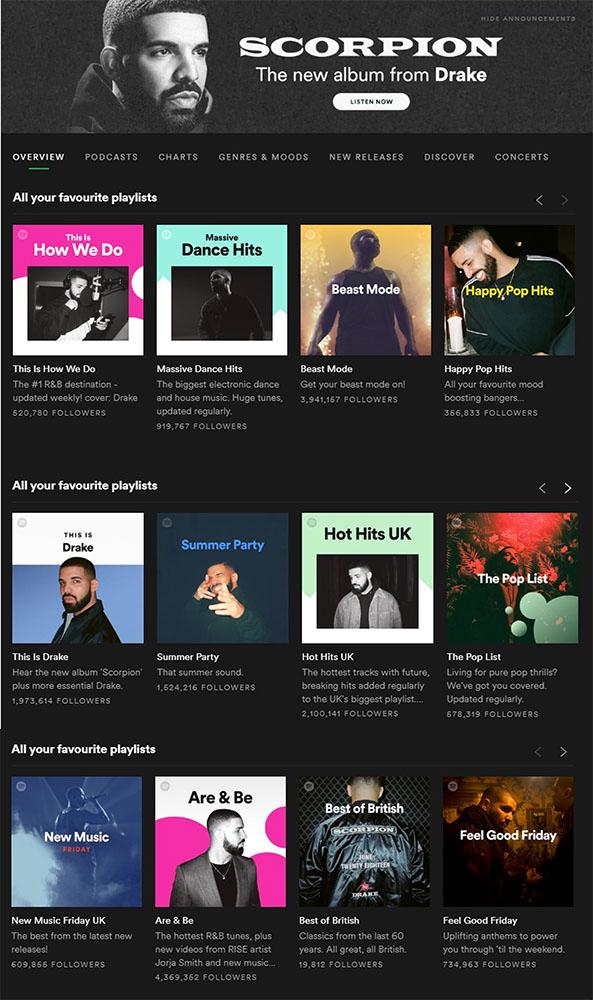The image showcases Drake's new album, "Scorpion," prominently featured on a sleek, modern digital music platform. The album title is visibly written in white font at the top against a dark background, giving it a striking contrast. Beneath this title, there is a visually engaging "Listen Now" button, encouraging immediate engagement. A photo of Drake, a Black man with neatly cropped short hair, a mustache, and a beard, is displayed prominently, drawing focus to the artist himself.

Below Drake's image, the navigation panel includes options such as Overview, Podcast, Charts, Genres & Moods, New Releases, Discover, and Concerts. The Overview tab is highlighted with a white background and a green underline, indicating it is currently selected. The main content area features a section labeled "All Your Favorite Playlists," organized into two visible rows, while a third row is partially obscured.

The first row includes four distinct playlists from left to right: "This Is How We Do," "Massive Dance Hits," "Beast Mode," and "Happy Pop Hits." The second row features playlists titled "This Is Drake," "Summer Party," "Hot Hits UK," and "The Pop List." Each playlist is tailored to different musical tastes and moods, providing a variety of listening options for fans.